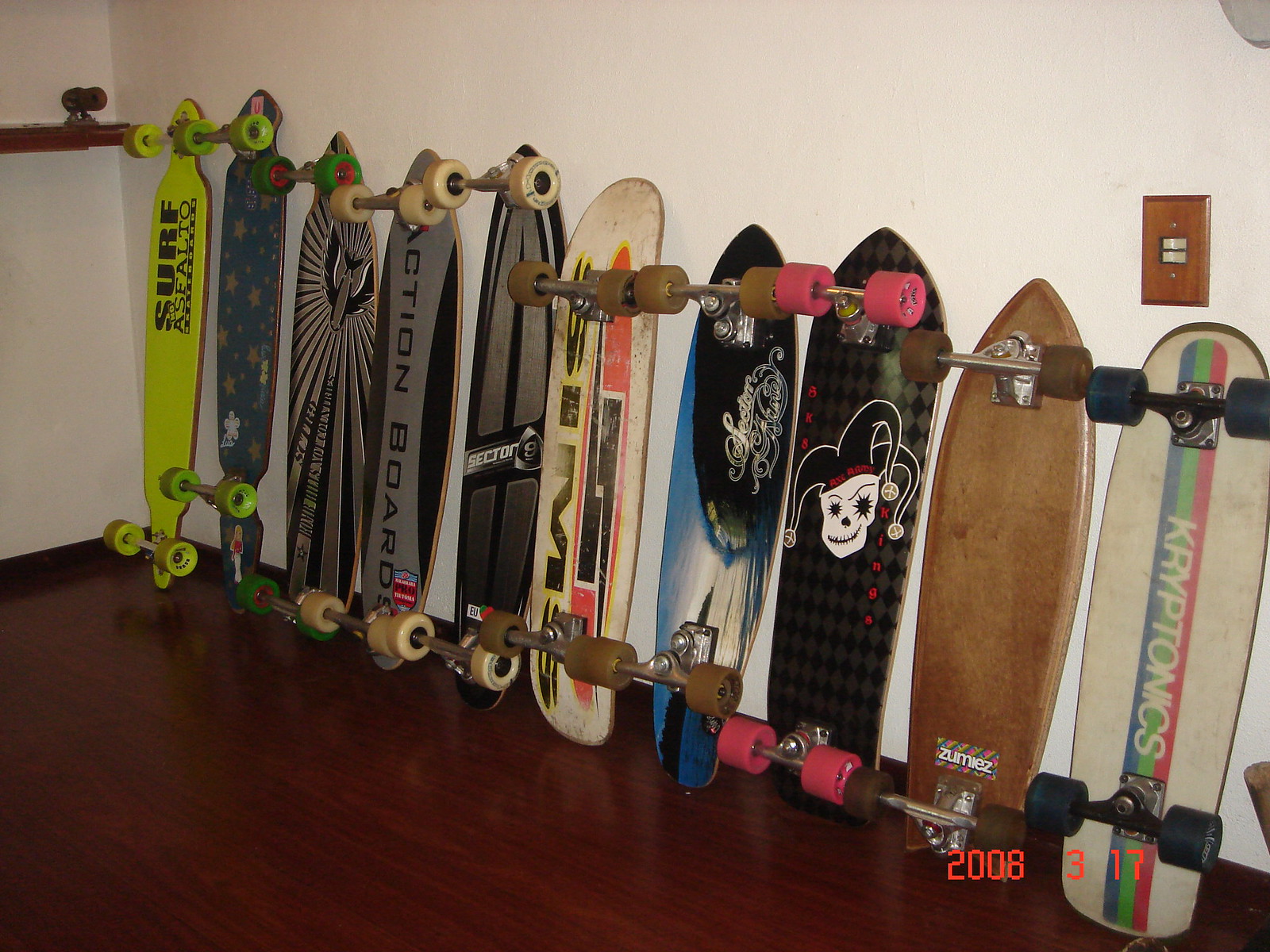The image features a neatly arranged collection of ten skateboards, all leaning vertically against a white wall in what appears to be a bedroom. The room has polished dark brown wooden floors, setting a contrasting backdrop for the array of skateboards that stand out with their varied designs. Here’s a detailed look at each skateboard from left to right: 

1. The first skateboard is a striking lime green with the partially legible text "Surf Asphalto," and is equipped with lime green wheels.
2. Next is a blue skateboard adorned with a colorful star pattern and matching lime green wheels.
3. The third board features a missile graphic in silver, emitting black and white lines reminiscent of sun rays, and it also has green wheels.
4. The fourth skateboard bears the phrase "Action Board" in black lettering, surrounded by silver and black elements, and is fitted with beige wheels.
5. The fifth board displays "Section Nine" in prominent white letters on a silver and black base.
6. A vibrant multi-colored skateboard follows, with what appears to be "Sims" written in black ink bordered in yellow on a white background, complemented by a black and red logo.
7. The seventh skateboard has a more complex design with black and blue sections, and possibly says “Gesture” in black or silver; it has brown wheels.
8. Following that is a board featuring a ghoulish jester with a skull face, set against a black background, and it has red wheels.
9. The ninth skateboard has a rustic wooden appearance, akin to an ironing board, with a Zumez sticker and distinctive brown wheels.
10. Lastly, a white skateboard with a blue, green, and red stripe running down the center, bearing the name "Kryptonix," finishes the lineup. This board is equipped with black wheels.

A light switch with a brown wood plate is also visible on the wall, adding a touch of homeliness to the scene. Additionally, a date stamp on the picture reads March 17, 2008.